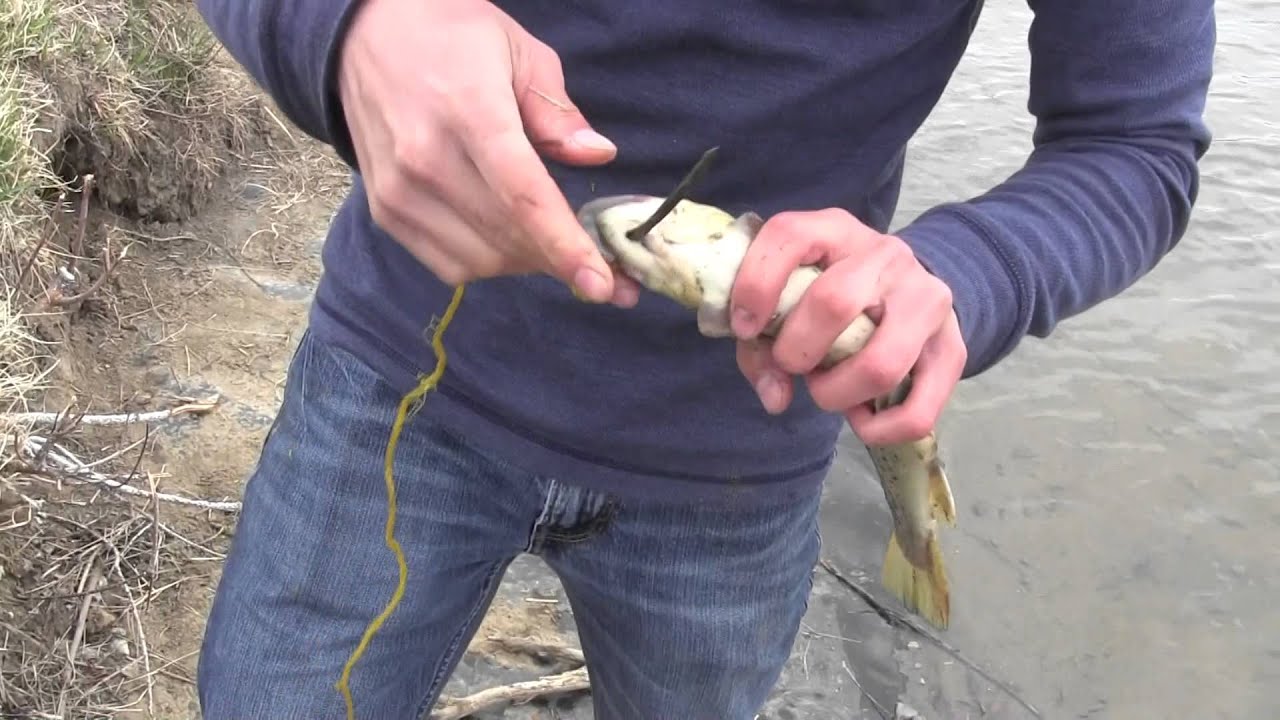In the image, a man, captured from the chest down to the knees, stands by a murky lake shore. He's donning a long-sleeve navy blue t-shirt and blue jeans. The cloudy day sets a somber tone over the brownish-gray waters, adding to the scene's muted palette. The ground is a mix of dirt and sparse grass, elevating slightly from the water's edge. The man grips a fish in his left hand, identifiable as a bullhead or catfish, with a visible yellow string hanging from his right hand. The fish, around eight or nine inches long, has a black hook about an inch and a half in size embedded in its underside mouth area. The man appears to be in the process of removing the hook, his right hand hovering close to the fish, enacting the careful process under the morning or afternoon light that highlights his hands and the fish against the murky backdrop.